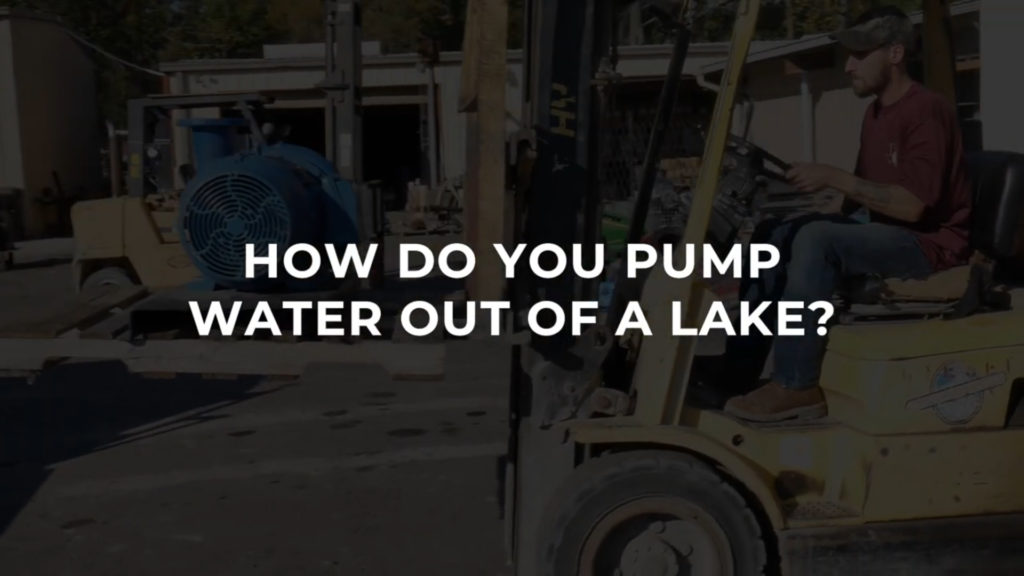The image features a slightly darkened scene to emphasize the central text, which reads in large white, capital letters: "HOW DO YOU PUMP WATER OUT OF A LAKE?" Situated in front of an open garage door, a bearded man in a gray baseball cap, maroon shirt, blue jeans, and working boots is operating a yellow forklift. The man, who appears to be wearing sunglasses, is positioned on the right side of the image, driving the forklift with his hands on the steering wheel. The forklift has a logo resembling a globe with a ring around it. In the background to the left, two large blue fans are visible, suggesting an industrial or construction setting. Smaller trucks are also scattered around, enhancing the busy, work-focused atmosphere of the scene. The darkened background contrasts with the bright white text, drawing viewers' attention to the question posed at the center of the image.